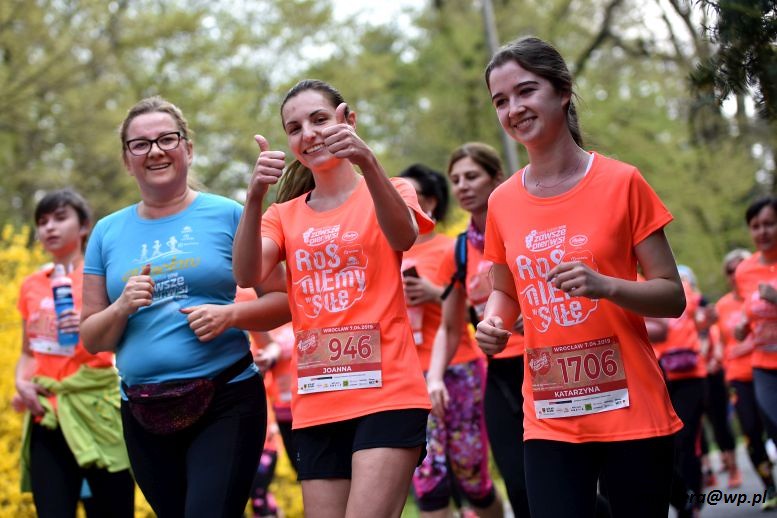In this vibrant outdoor image, a group of people, predominantly women of various ages, are participating in what appears to be a running event, likely a 5K race. Central to the image are three women, each exuding a sense of camaraderie and enthusiasm. The woman on the left, wearing glasses, sports a light blue t-shirt, black trousers, and a fanny pack. The woman in the middle, identified as Joanna, is energetically giving two thumbs up, dressed in an orange t-shirt with the race number 946 and short black shorts. The scene captures her exuberance. Next to her is Katarzyna, smiling with her brown hair pulled back; she too wears an orange t-shirt, dark trousers, and the race number 1706. Both women's bibs prominently display their names. The backdrop features the lush greenery of trees, lending a refreshing ambiance to the event. Other participants are visible in the background, slightly blurred, enhancing the sense of a bustling and lively group activity. Text in the image reads "Rosnably Sweet," and a partially visible link with "wp.pl" suggests that this event is likely outside the United States. The overall scene is invigorating, capturing the spirit of a communal race event.